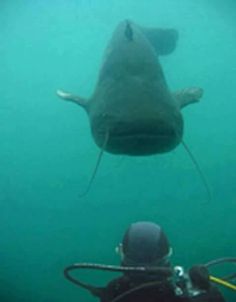In the image, a scuba diver, clad in black gear including a black helmet or skull cap, goggles, a regulator, and a tank on his back, is positioned at the bottom right corner. The water surrounding him is a murky gradient, transitioning from a lighter blue at the top to a deeper, darker blue towards the bottom. He's gazing upward towards an enormous catfish, which seems almost as large as he is, although the perspective exaggerates its size. The catfish, grey in color with prominent whiskers, a flat mouth, and lateral fins extended to each side, is approaching from above. Its long fin tail stretches out towards the upper right corner of the image. If the scuba diver and the catfish continue on their current trajectories, a head-on collision seems imminent. The contrast between the scuba diver's gear and the catfish's imposing presence accentuates the surreal, underwater encounter.